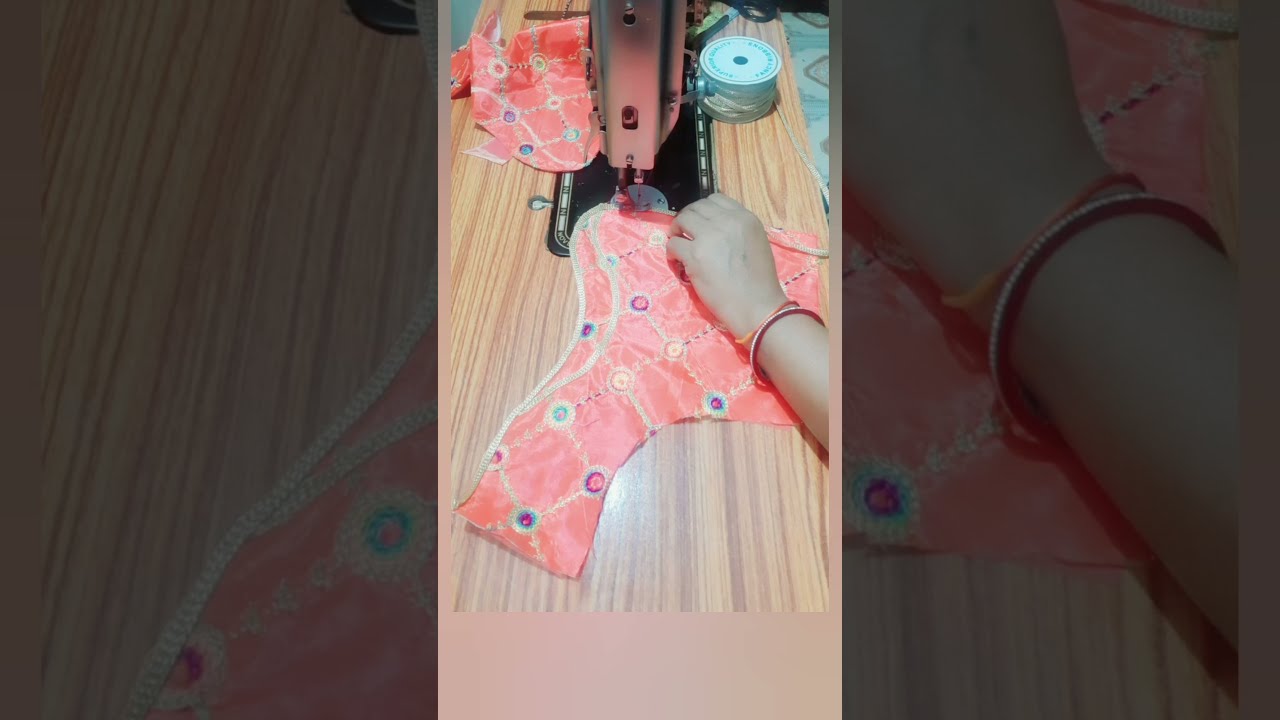The photograph captures a detailed close-up of a woman sewing on an industrial black and silver sewing machine with a wooden base. The scene is presented in portrait orientation with a darkened, blurred background of the same image in landscape. The woman's light-skinned left hand, adorned with two bracelets, is guiding a peach-colored fabric featuring an array of vibrant, multicolored circles and squiggly lines in red, yellow, blue, and green. The sewing machine is engaged with the edge of this fabric, possibly piecing it with another segment visible behind the machine. The table on which the sewing machine rests has a light wood grain surface, and a roll of ribbon or trim is positioned to the right side of the machine, further adding to the authentic sewing environment.